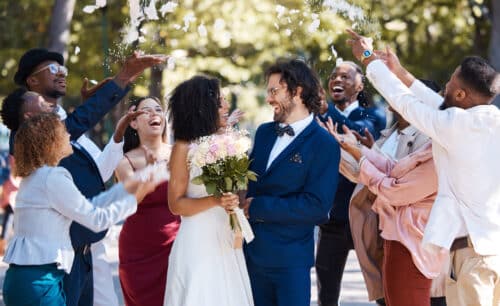A joyful couple, newly married, stands at the center of this sunny, outdoor scene, set against a backdrop of lush green trees with sunlight filtering through. The groom, sporting glasses, medium-length unkempt hair, and a messy beard, is dressed in a dark blue tuxedo with a bow tie. Beside him, the radiant bride, with natural hair texture, wears a sleeveless white dress – its simplicity and elegance accentuated by a fitted bodice and flowing skirt. She holds a vivid bouquet of purple, pink, and white flowers. Surrounding the couple, their casually dressed friends celebrate by throwing biodegradable confetti into the air, their joyous expressions mirroring the couple’s bright smiles as they gaze lovingly at each other. Among the friends, a girl in a red dress is seen clapping joyously. They all stand on a sidewalk, with the vibrant greens of trees encircling the happy scene of this laid-back wedding day.